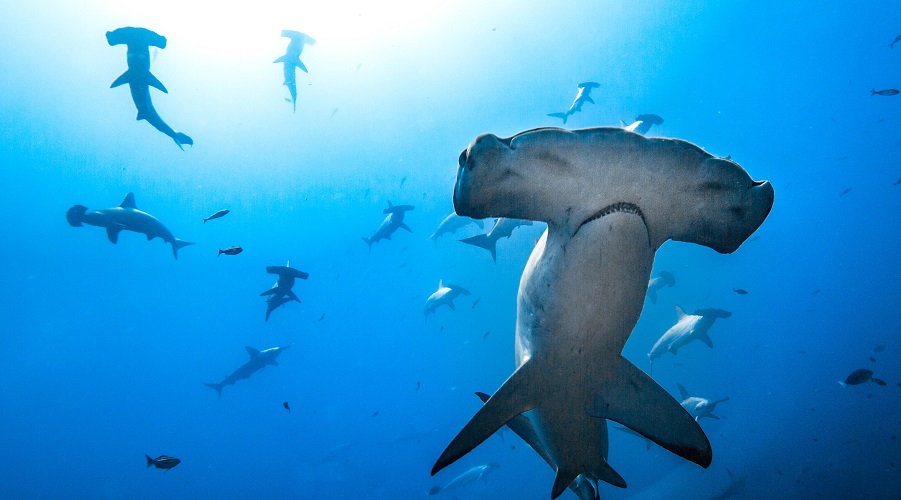An underwater scene reveals a dynamic array of fish dominated by numerous hammerhead sharks. In the foreground, an up-close and slightly offset view of a hammerhead shark captures attention. The shark has a distinct light gray or white underbelly, contrasting with its darker gray sides. Its head extends outward on either side into a T-shape, ornamented with blue edges and wavy lines on top. Its curved, crescent-moon-shaped mouth is filled with small, sharp white teeth, and its lateral fins and large tail are visible. The vibrant blue water, shimmering with sunlight from above and darkening into deeper shades below, serves as the backdrop for a multitude of other hammerhead sharks, some of which appear to circle the area, creating a sense of depth and movement in this vivid marine environment.